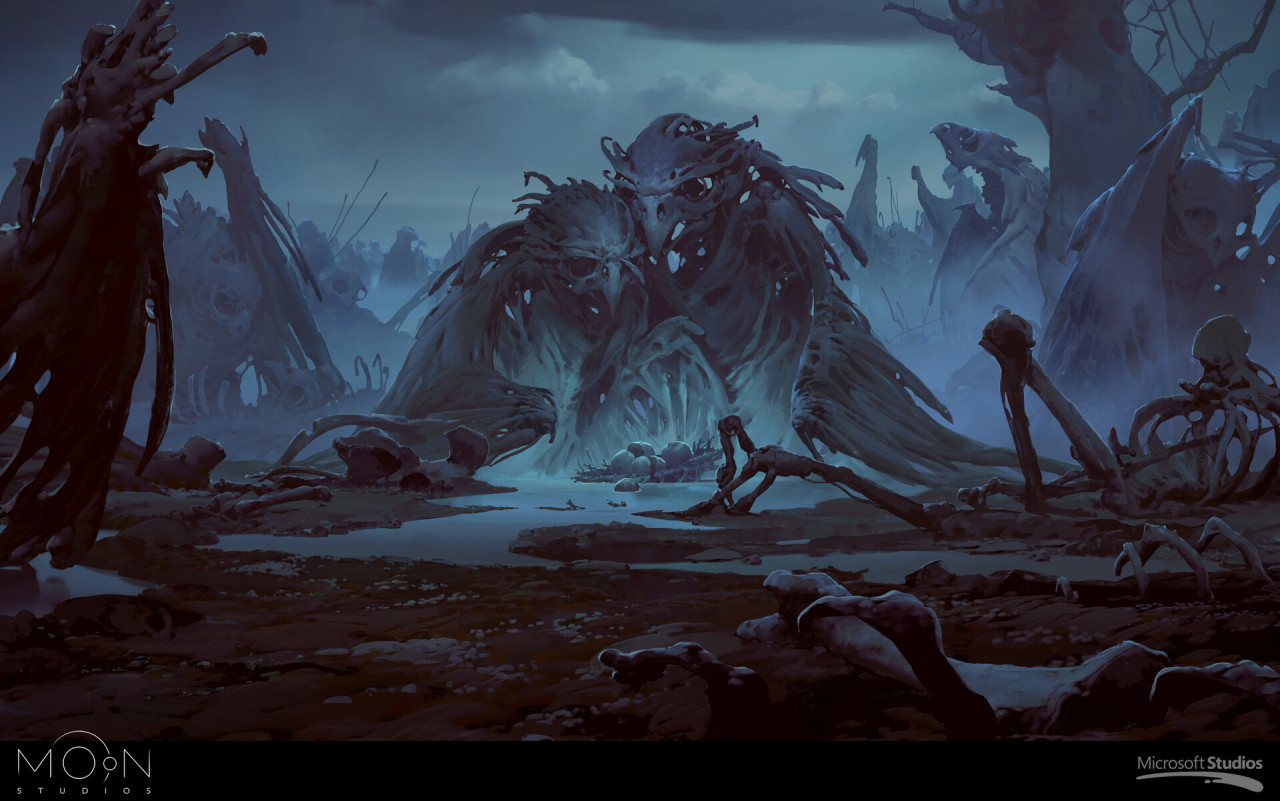The image portrays a desolate and ominous swamp scene bathed in deep navy, turquoise, and various shades of dark blue, evoking a pitch-black night in a forest. Surrounding the scene are bent, leafless, dead trees, adding to the eerie atmosphere. At the center of the image, two large skeletal figures, resembling giant bird skeletons, are huddled together, possibly forming a shelter. They appear to be examining something on the ground amid a greenish light, resembling rocks or perhaps hatched eggs, which are faintly illuminated as if by a hidden fire. The surrounding area is littered with bones and other skeletal remains, contributing to the scene’s sense of decay and desolation, enhanced by small puddles and a dirt surface. The overall atmosphere is suggestive of a post-apocalyptic world, where toxic air and a sense of devastation dominate. Written in the corners are the names "Moon Studios" and "Microsoft Studios."